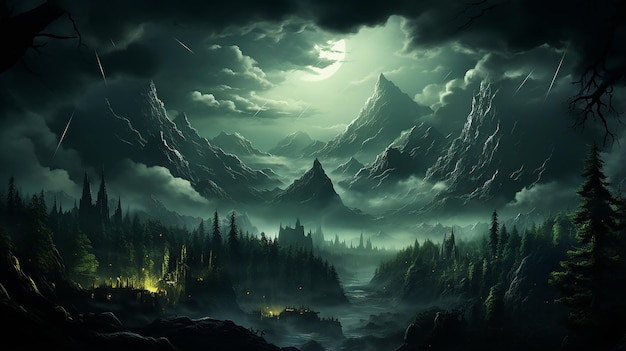This digital painting depicts a hauntingly beautiful, gloomy outdoor landscape. Dominated by dark greens and blacks, the scene is filled with towering pine trees, jagged mountain peaks, and swirling, ominous clouds. The moon glows faintly, casting an eerie light over the foggy terrain, which includes a meandering river flowing through the center. In the lower left corner, the dim flicker of a fire provides a stark contrast to the overall darkness, possibly from a secluded campsite or small structure. The image feels damp and dreary, evoking a spooky atmosphere reminiscent of a Halloween night. Subtle tinges of blue and yellow pierce through the monochrome setting, adding depth and mystique to the scene.